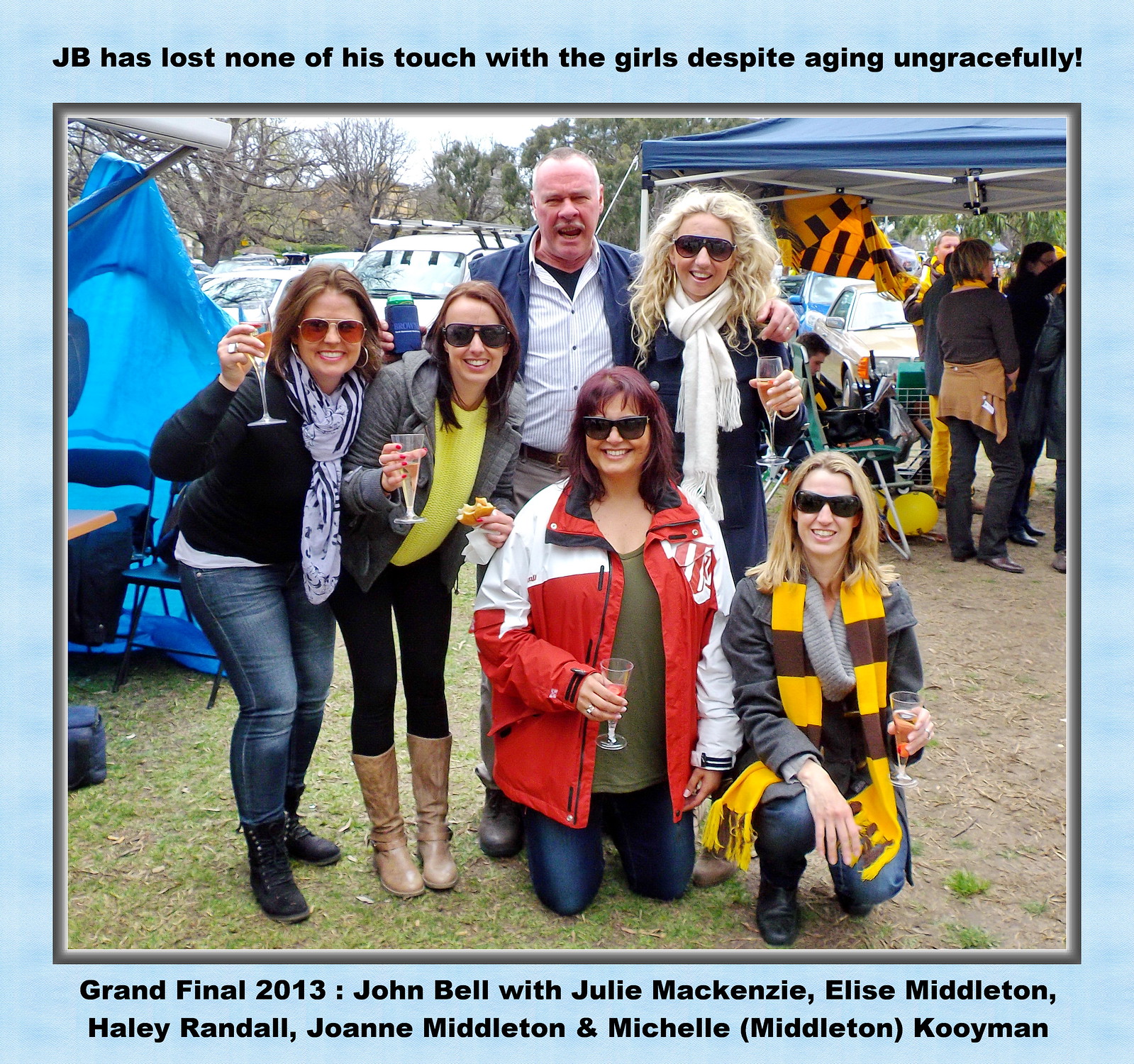In the image, we see a jubilant outdoor gathering where an older gentleman, likely John Bell (referred to as JB), stands among five women on a grassy lawn. The group is energetically raising their champagne glasses in a celebratory toast towards the camera, suggesting a moment of shared festivity. Two of the women are kneeling in front, while the man and the other women stand behind. The women's ages range from their 20s to 30s, and they are all dressed warmly in coats and scarves, implying a chilly day. JB, appearing to be in his 50s, sports a blue jacket and a white shirt and has his left arm around the nearest woman who is wearing sunglasses and a white scarf.

In the surroundings, the backdrop features a blue tent with several people visible beneath it and various vehicles, adding to the sense of a tailgating or sporting event atmosphere. This is reinforced by the blue border around the image, with the top text reading, "JB has lost none of his touch with the girls despite aging ungracefully," and the bottom text stating, "Grand Final 2013," along with the names: John Bell, Julie McKenzie, Eliza Middleton, Haley Randall, Joan Middleton, and Michelle Middleton-Kumian. The scenic setting also includes some trees and what appears to be a camper or bus, adding context to this spirited outdoor celebration.